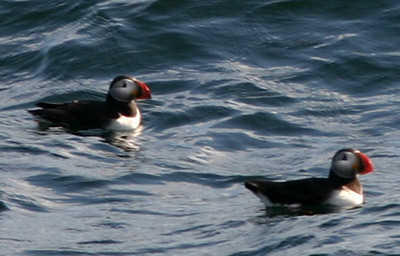In this image, two puffins float on slightly choppy, icy blue-gray ocean water. The first puffin is positioned towards the left-middle of the frame, while the second is in the lower right corner, both facing to the right. Their distinct orange beaks, one notably tipped with black, stand out against the cold backdrop. These puffins feature black plumage on the top of their heads, which extends down their backs in a semi-circular shape, contrasting sharply with the white of their chests and the area around their black eyes. Their straight backs and barely visible wingtips add to their streamlined appearance. The lighting in the scene suggests it is either early morning or late afternoon, as there is a subdued, indirect light reflecting off the water’s slightly rippled surface. The ocean appears somewhat rough, giving the impression of potentially challenging swimming conditions for the birds.